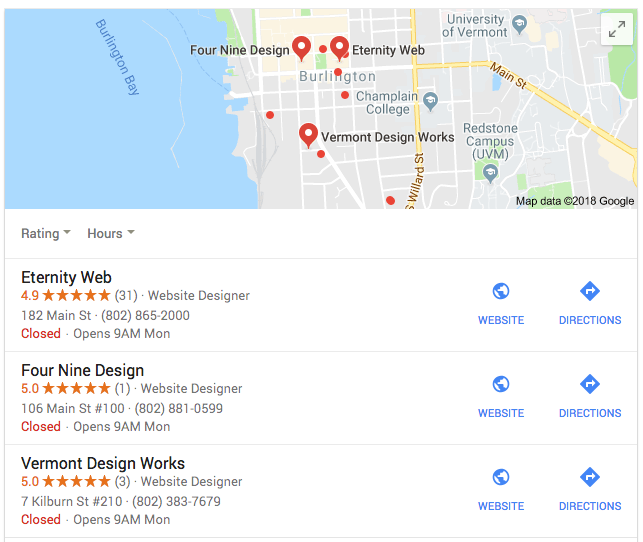This image displays a Google search results page specifically focused on location-based results in Vermont. Dominating the top portion of the screen is a light gray map showcasing a segment of Vermont, highlighted with roads and streets in white, while the main roads are marked in light yellow with black text labels. Red location icons pinpoint four business locations on the map. Burlington Bay, a prominent body of water, is situated to the left of this area.

Beneath the map, there's a vertical list featuring businesses in the region. Each listing provides essential details such as operating hours, contact numbers, and star ratings. To the right of each business entry, there are two icons: a bright blue globe indicating a link to the website and a diamond shape with a white arrow labeled "directions."

The first listed business is "Eternity Web," shown in bold black text. Complementing its name, there is a 4.9-star rating displayed in dark orange. Below the rating, gray text describes the business as a "Website Designer," followed by its address "182 Main Street," and its phone number "802-865-2000." Two additional businesses, "49 Design" and "Vermont Design Works," are similarly listed below Eternity Web, each in black text.